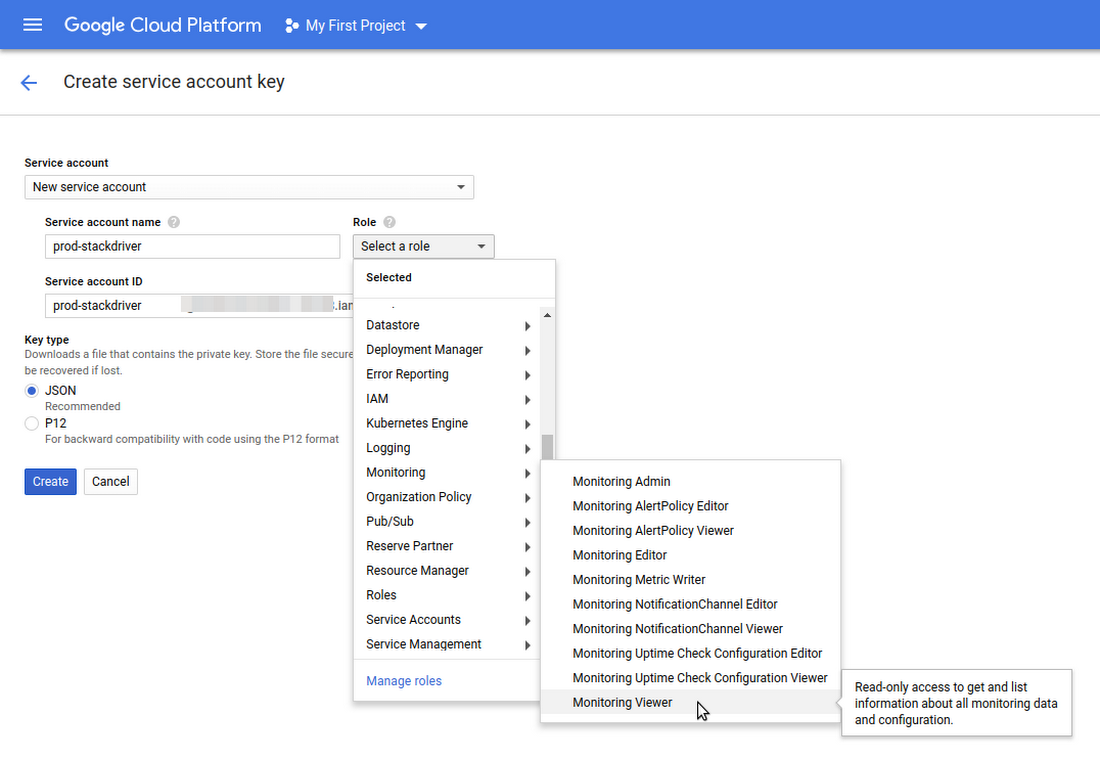The screenshot displays a Google Cloud Platform interface, primarily featuring a clean white background with black text. Dominating the top of the screen is a blue menu bar. On the left side of this bar, three white lines indicate a clickable menu option, followed by the "Google Cloud Platform" label in white text. Adjacent to this is "My First Project" accompanied by a drop-down arrow.

Beneath this bar on the left, there is a left-pointing blue arrow next to the text "Create Service Account Key" in black. Below this, the label "Service Account" appears with a corresponding drop-down menu displaying "New Service Account" as the chosen option.

The interface next highlights "Service Account Name" with an input field filled with the text "Prod Stackdriver." Further down, the label "Role" is followed by a drop-down menu that initially reads "Select a Role."

The menu expands into a three-window cascade. The first window, titled "Selected," lists options like Data Store, Deployment Manager, Error Reporting, IAM, Kubernetes Engine, Logging, Monitoring, and Organization Policy. From this list, the window for "Monitoring" reveals its own set of roles in the next window titled "Managed Roles," including "Monitoring Admin," "Monitoring Alert Policy Editor," "Monitoring Editor," and "Monitoring Viewer." "Monitoring Viewer" is selected, prompting a pop-up that explains: "Read Only Access to get endless information about all monitoring data and configuration."

Overall, the screenshot captures the detailed process of configuring a new service account key within the Google Cloud Platform, emphasizing the steps involved in setting roles and permissions.